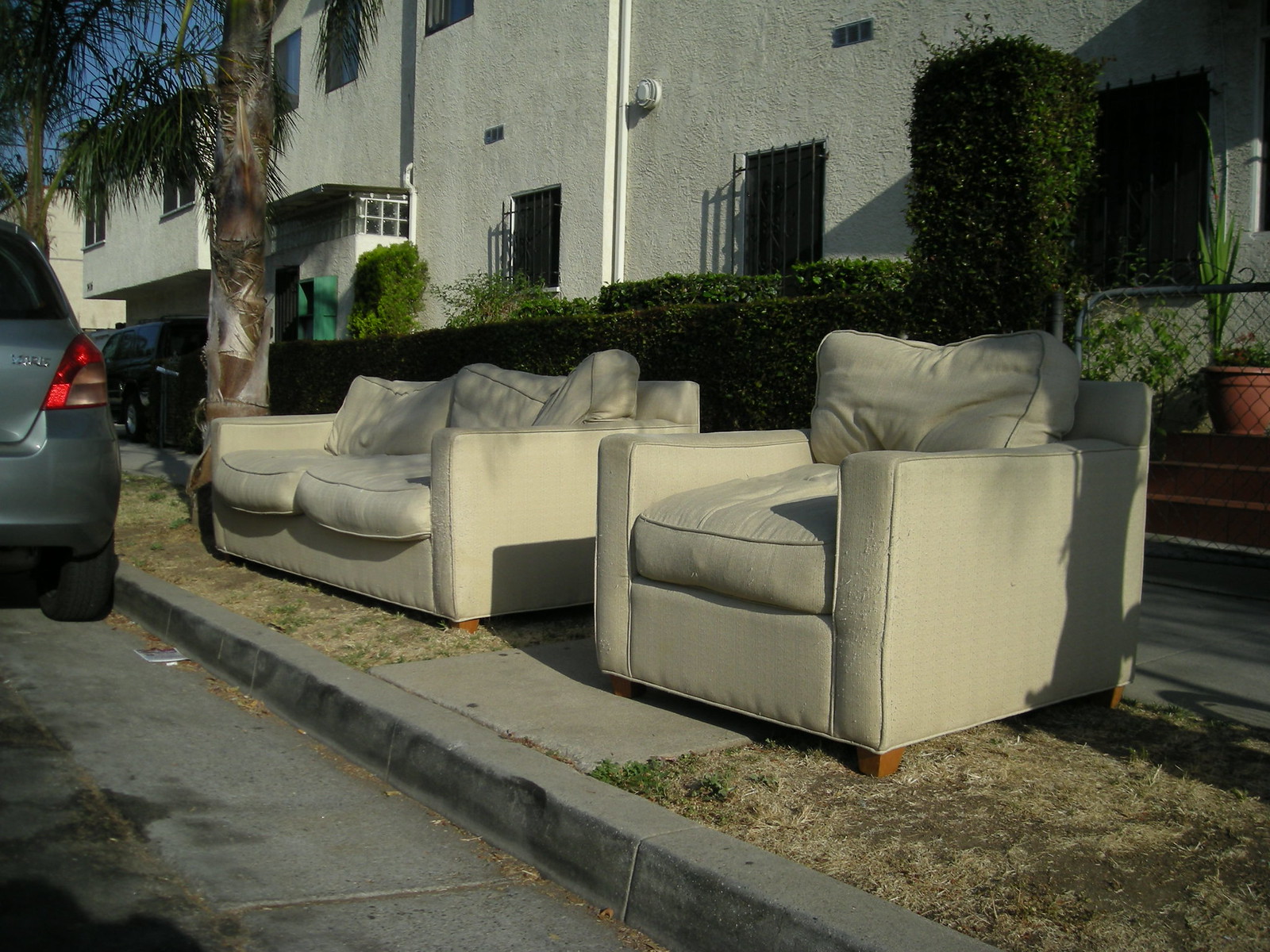The image captures a city street scene with a well-worn light green loveseat and chair (possibly tan or off-white) positioned on patches of dead grass between the curb and sidewalk. The furniture, which shows signs of use such as cat scratches, features fluffy seat and back pillows, and brown wooden stands. Adjacent to the loveseat, a tree casts its shadow, adding depth to the outdoor setting. Directly behind the chair, a tall fence borders a hedge, and beyond that, a white stucco building with barred windows and doors. A walkway leads past potted plants up to the building, completing the urban snapshot.